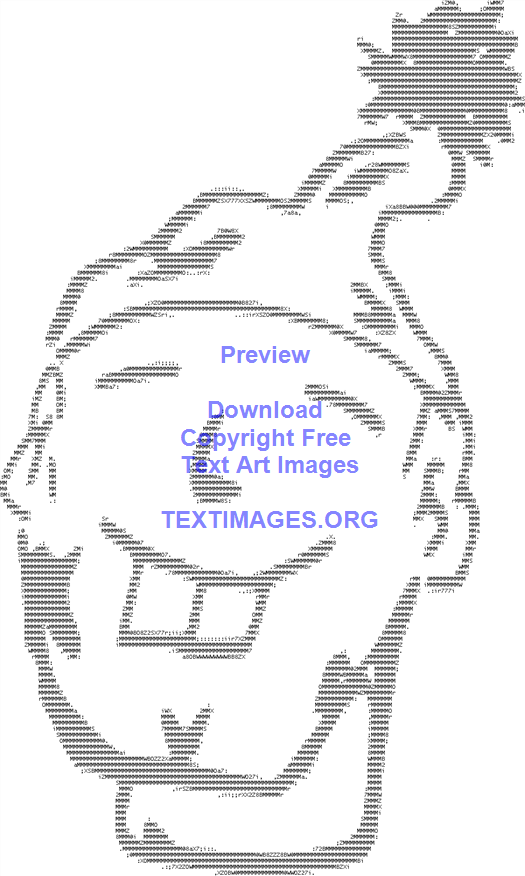The image features a simplistic, computer-generated cartoon drawing of a man's head and neck created with text art, reminiscent of old-fashioned dot matrix or bubble jet printers. The man's face is defined using various keyboard characters, including question marks and the letter 'M.' He has a lighthearted expression, characterized by a wide grin that exposes two large front teeth. His eyes are closed in a joyful manner, and he wears a distinctive hat that resembles an elf's, complete with a floppy shape and a pom-pom at the tip. The background is plain white. Above the figure, blue text is sequentially arranged in individual lines, reading: "Preview," "Download," "Copyright free," "Text art images," and "textimages.org." The overall impression is that of a cheerful, whimsical character brought to life through the nostalgic art of keyboard symbols.